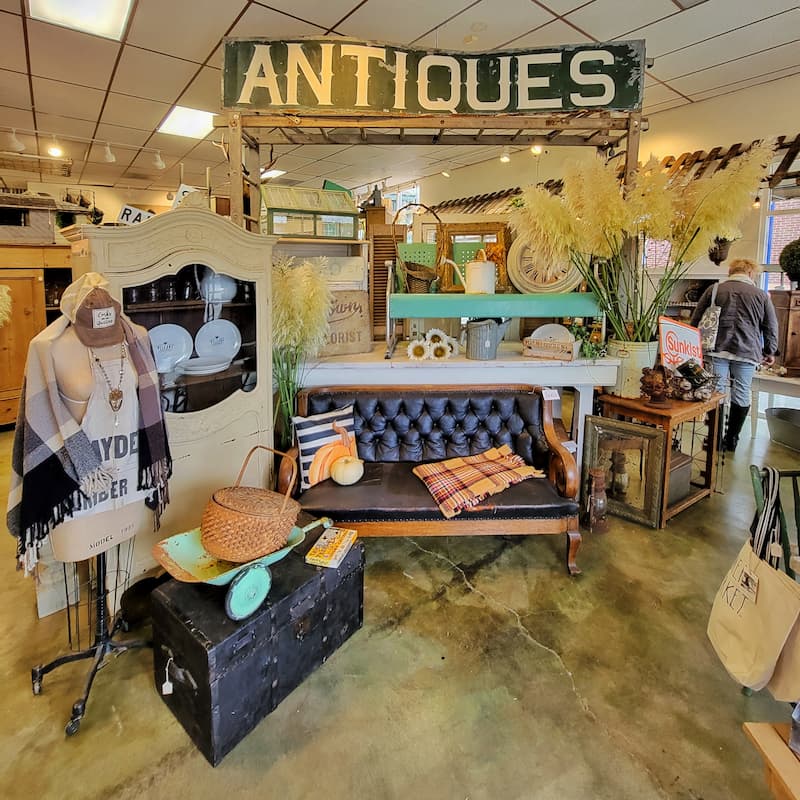The image depicts a quaint and nostalgic scene inside an antique store, characterized by its aged ambiance and eclectic collection of treasures. The store has a cream-colored drop ceiling with lit square panels and fluorescent lights, casting a warm glow over the slightly discolored and cracked concrete floor. Dominating the center of the photograph is a creative display made from old wooden ladders. At the top of this display, a sign made of green, weathered wood reads "ANTIQUES" in cream letters, immediately drawing attention.

Below the sign sits an old leather loveseat settee adorned with a mix of decorative throw pillows, including a black-and-white striped one and another in plaid, along with a small white pumpkin. Next to the loveseat, a vintage black metal chest serves as both a functional piece and a decorative item, topped with a turquoise planting basket that holds a wicker basket. A headless mannequin dressed in a tank top, plaid shawl, baseball cap, pendant, and necklace adds a quirky touch to the display. 

Behind the mannequin and loveseat, there is a white china hutch with open front glass doors, showcasing an array of white china plates. Visibly peeking from the far background, a figure with their back to the camera seems to be engrossed in exploring the various items scattered around the store, adding to the lively atmosphere of this charming antique shop.